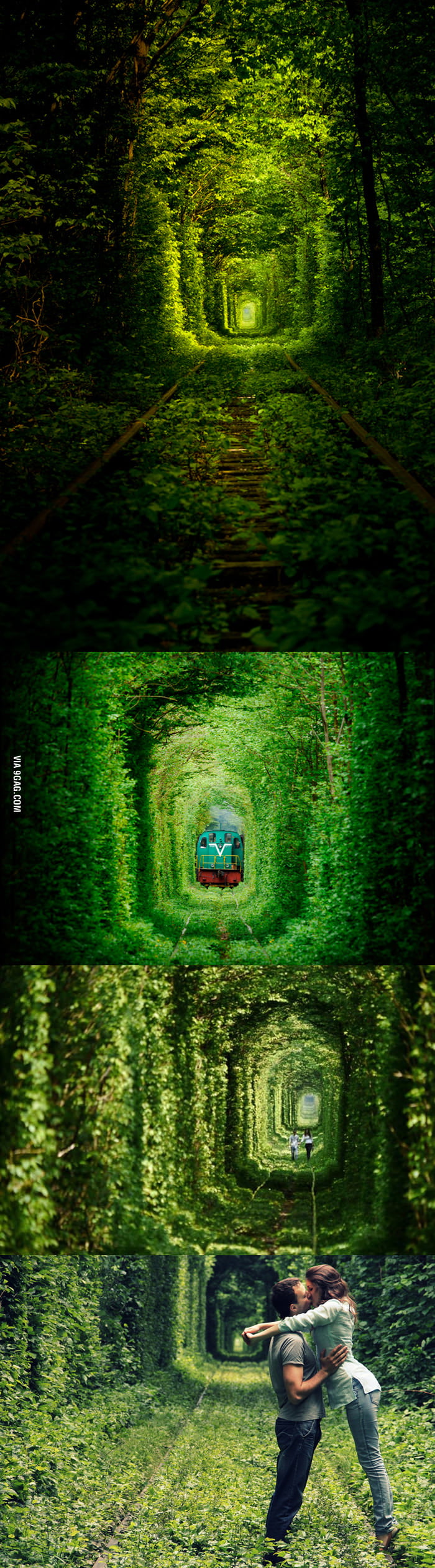This vertical photo collage consists of four distinct panels stacked on top of each other, each capturing a segment of a lush, forested railway tunnel. The dense greenery forms concentric rectangular frames, drawing the viewer's eye deep into the woodland path.

The top image of the collage is dark, showcasing an old railway track overgrown with vegetation. As the image extends into the background, it gradually becomes lighter, emphasizing the depth of the forest. The second image, slightly brighter and with a green hue, features a distant train traveling through the tunnel of trees. This panel bears a small watermark on the left side that reads "via 9gag.com" in white text.

The third image shifts the focus to a more intimate scene where two people are seen walking along the railway track, enveloped by the surrounding forest. These figures face away from the camera, moving towards the vanishing point of the composition.

The final, bottommost panel zooms in on a tender moment between a couple. The man, dressed in a gray t-shirt and blue jeans, embraces the woman, who is slightly elevated on a ledge. She wears a blue long-sleeve shirt and gray jeans, her arms lovingly draped around his neck as they share a kiss. This romantic tableau, set against the serene, green backdrop of the overgrown railway, captures a timeless moment of affection.